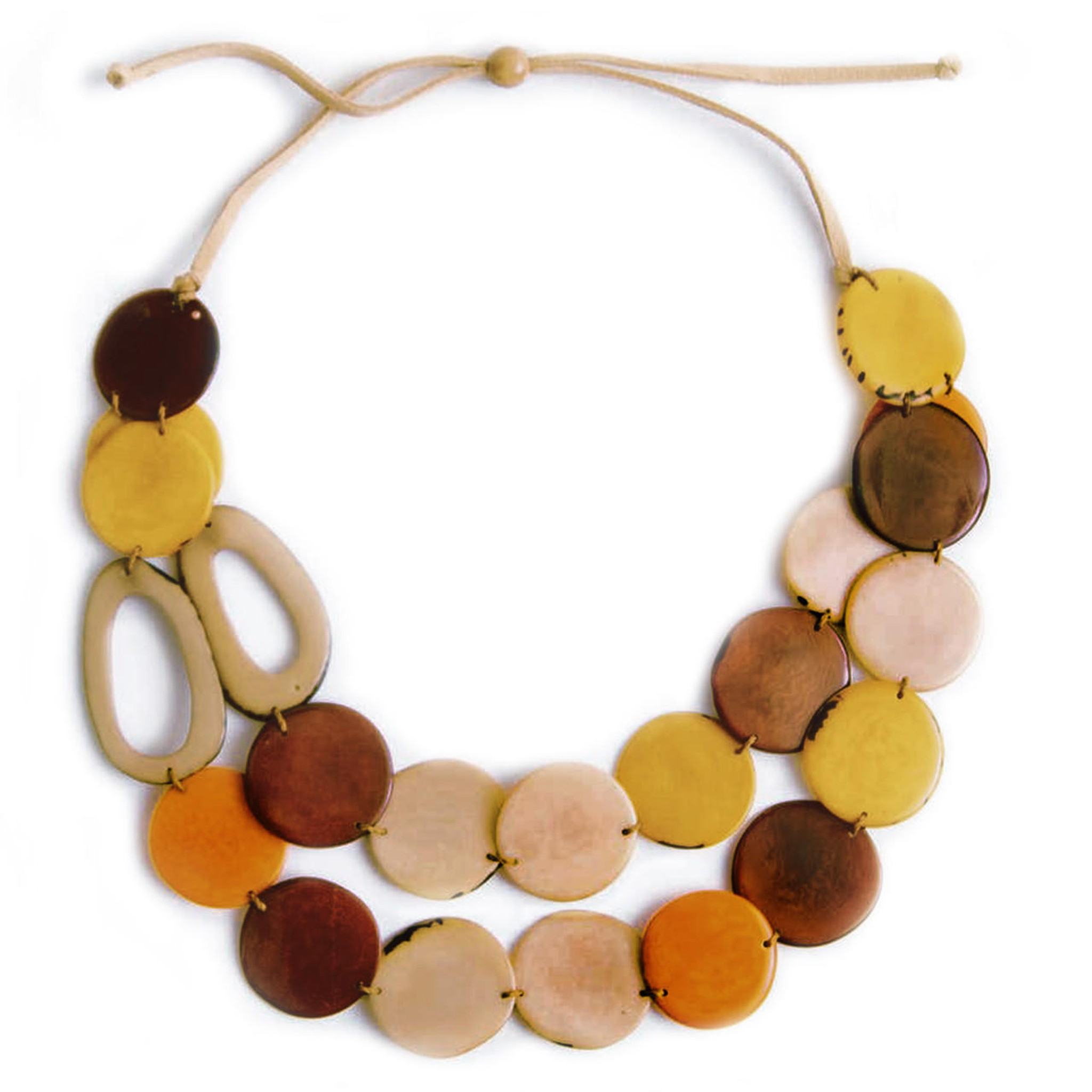This is a color photograph of a handcrafted necklace made from a pale brown leather or hemp cord tied at the top with a roundish knot. The necklace consists of several beads intricately arranged in a mostly circular pattern, focusing on the bottom three-fourths. A highlight feature is a small bead that serves as an adjustable clasp, enabling the necklace to be resized easily by pulling the ends of the cord through it. The beads are primarily round discs in various hues, including brown, dark brown, golden, orange, ivory, yellow, pale pink, and a sort of pale peach. Adding to its uniqueness, there are two notable oval-shaped, open-centered wooden or ceramic beads on the left, breaking the uniformity of the circular beads and adding a touch of asymmetry. The background of the photograph is plain and pale white, with no other objects or text visible.